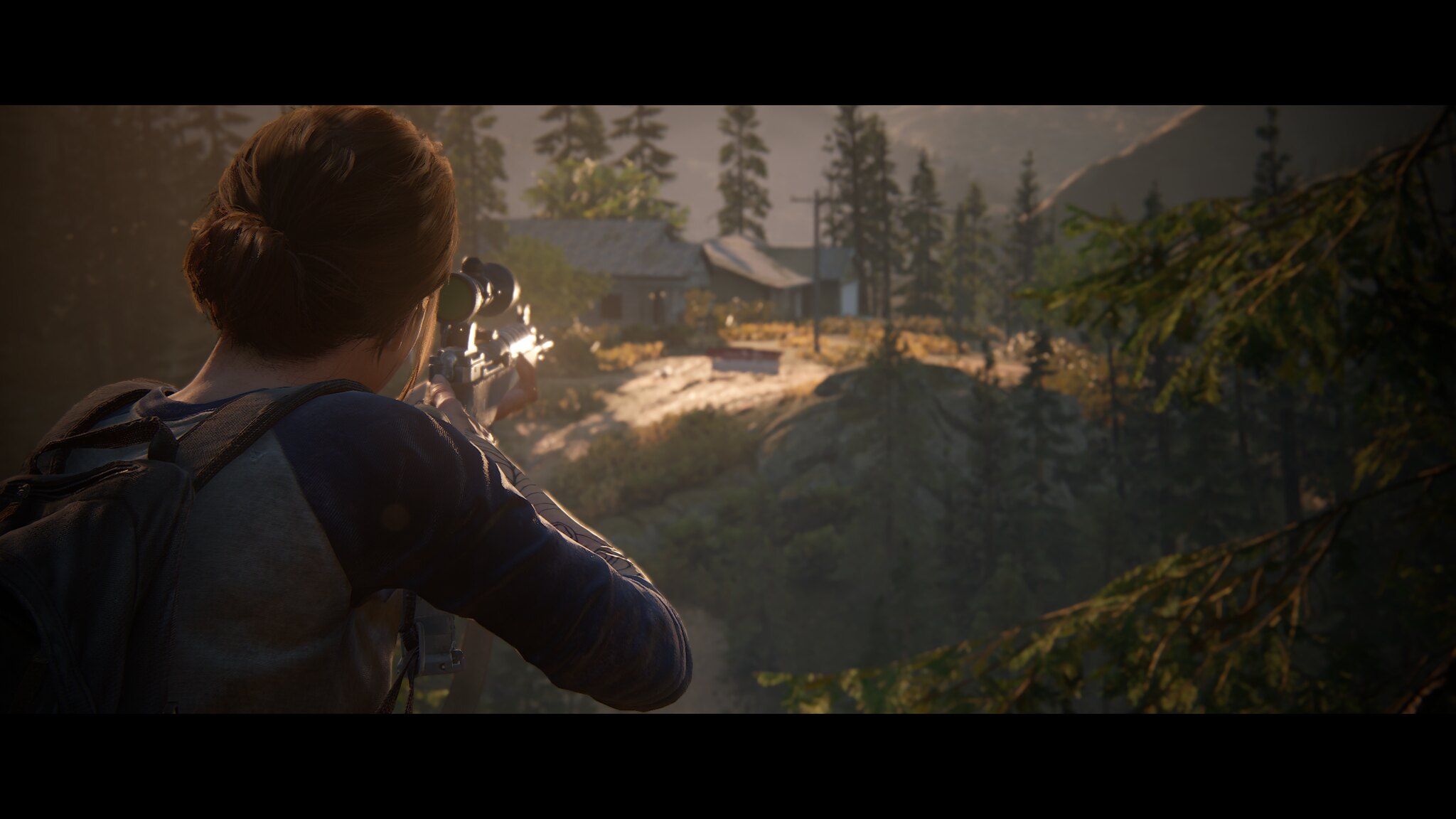A cinematic widescreen screenshot from a computer video game depicts a tense moment of action. The scene, framed by black borders at the top and bottom to enhance its cinematic feel, features a woman standing with her back to the viewer. She is holding a gun, strategically aiming it into the distance. The setting behind her is a picturesque, mountainous landscape dotted with tall, green trees and a few scattered houses. The mountains loom in the far distance, adding depth and grandeur to the scene. The woman appears to be taking aim at the distant houses, her stance and the gun in her hands suggesting a looming confrontation. The overall composition of the image captures a blend of natural beauty and impending action, evoking a sense of anticipation and drama.